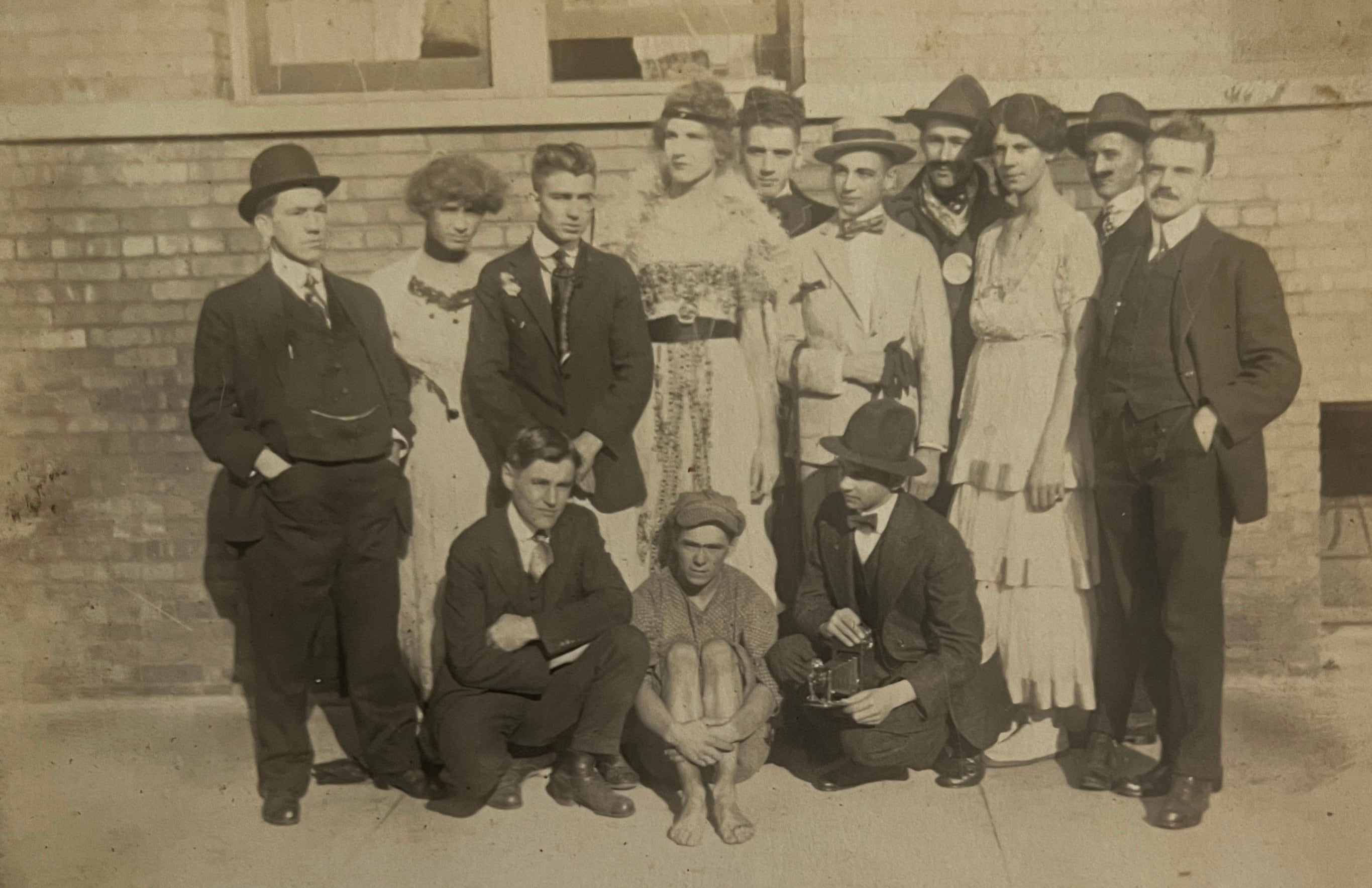This is an old, worn black, white, and gray photograph depicting a group of 13 individuals, likely taken in the 1920s. They are standing and sitting on a concrete sidewalk in front of a brick building with windows visible just above their heads. The group consists of 10 men and 3 women, the majority of whom are standing while three are either kneeling or sitting in front. The men are predominantly dressed in well-to-do, dark suits with ties, some adorned with top hats and chain accessories. One stands out in a distinct white suit, bow tie, and straw hat. The women are dressed like flappers, with headbands and frilly dresses, indicative of the era. Among them, one individual, possibly a young person, kneels with their knees curled to their chest, wearing a cap and less formal attire, including shorts and no shoes or socks, suggesting a different social standing. Most of the group gaze directly at the camera while a few look elsewhere. All individuals appear to be white-skinned.